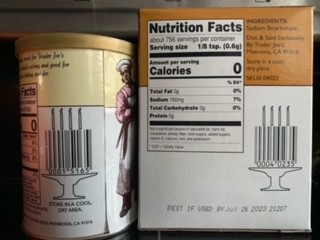In this image, we see two different products side by side. Both containers display nutritional facts and other product information. The container on the left is cylindrical with a gold plastic cap and a label featuring a yellow stripe at the top and a white bottom. It depicts a chef wearing a pink shirt, a white apron, and a white chef's hat. There is also a barcode visible on the cylindrical container.

Adjacent to this is a rectangular cardboard box. The top of the box is orange, and the bottom is white. It features an outline drawing of a birthday cake on a pedestal with four candles. The box has a "Best if used by July 26, 2023" label and displays nutritional information, including zero calories, zero total fat, 180 mg sodium, zero total carbohydrates, and zero protein per serving. The box also has another barcode and lists ingredients, though most of them are illegible except for sodium bicarbonate. The shared elements between both containers emphasize their nutritional facts and expiration date.